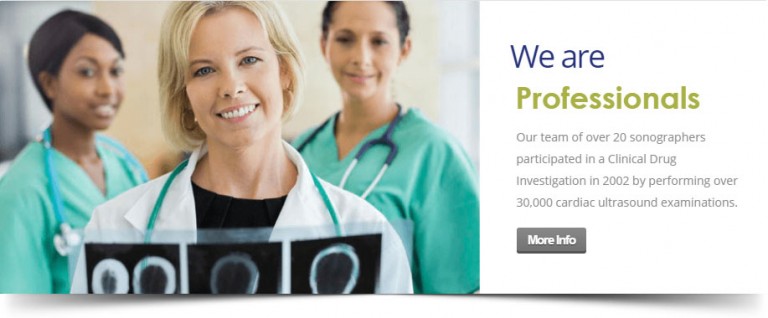This image is a screenshot of an online advertisement. On the left side of the advertisement are three medical professionals, each depicted in a clear and detailed manner. In the forefront stands a female doctor with short, chin-length blonde hair. She is smiling broadly, showing her teeth, and is wearing a black t-shirt under a white lab coat. She appears to be holding some x-rays in her hands. 

Behind her, slightly to the left, is a nurse dressed in light blue scrubs. She has brown skin, short black hair, and a light blue stethoscope draped around her shoulders and neck. She too is smiling, showing her teeth. 

To the right side in the image stands another medical professional, also wearing aqua blue scrubs, but with a navy blue stethoscope around her neck. She is smiling gently, though not showing her teeth, and has brown hair.

The advertisement text reads: "We are professionals" — with "We are" in blue and "professionals" in green. Below this, a detailed statement follows: "Our team of over 20 sonographers participated in a clinical drug investigation in 2002 by performing over 30,000 cardiac ultrasound examinations." 

At the bottom of the advertisement, there is a button labeled "More Info."